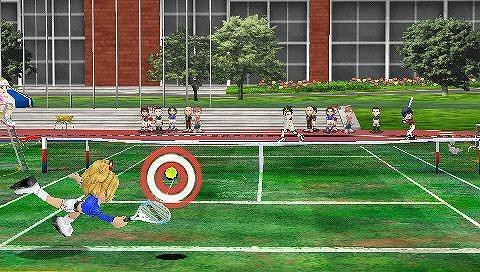The image appears to be a snapshot from a sports video game, depicting a vibrant tennis match. The scene is set on a green tennis court marked by white lines, with a dark net featuring a white border and a central white stripe. The foreground showcases a dynamic moment where a blonde-haired character, wearing a blue top, white shorts, and white shoes, lunges to hit a tennis ball with a racket. The ball is aimed at a red and white bullseye target, emphasizing precision.

In the background, there is a substantial building predominantly composed of glass and red brick. Surrounding the building are brick walls with multiple black-paned windows accented by white dividers. In front of this architecture lies a lush grassy field adorned with trees and a colorful flower bed. Additionally, white bleachers populated by spectators are visible.

Amidst the audience, a person on the far right intriguingly holds a baseball bat in a swinging motion, adding a unique element to the scene. On the left, a high chair accommodates a watcher overseeing the match, further enhancing the lively and detailed ambiance of this sports game image.